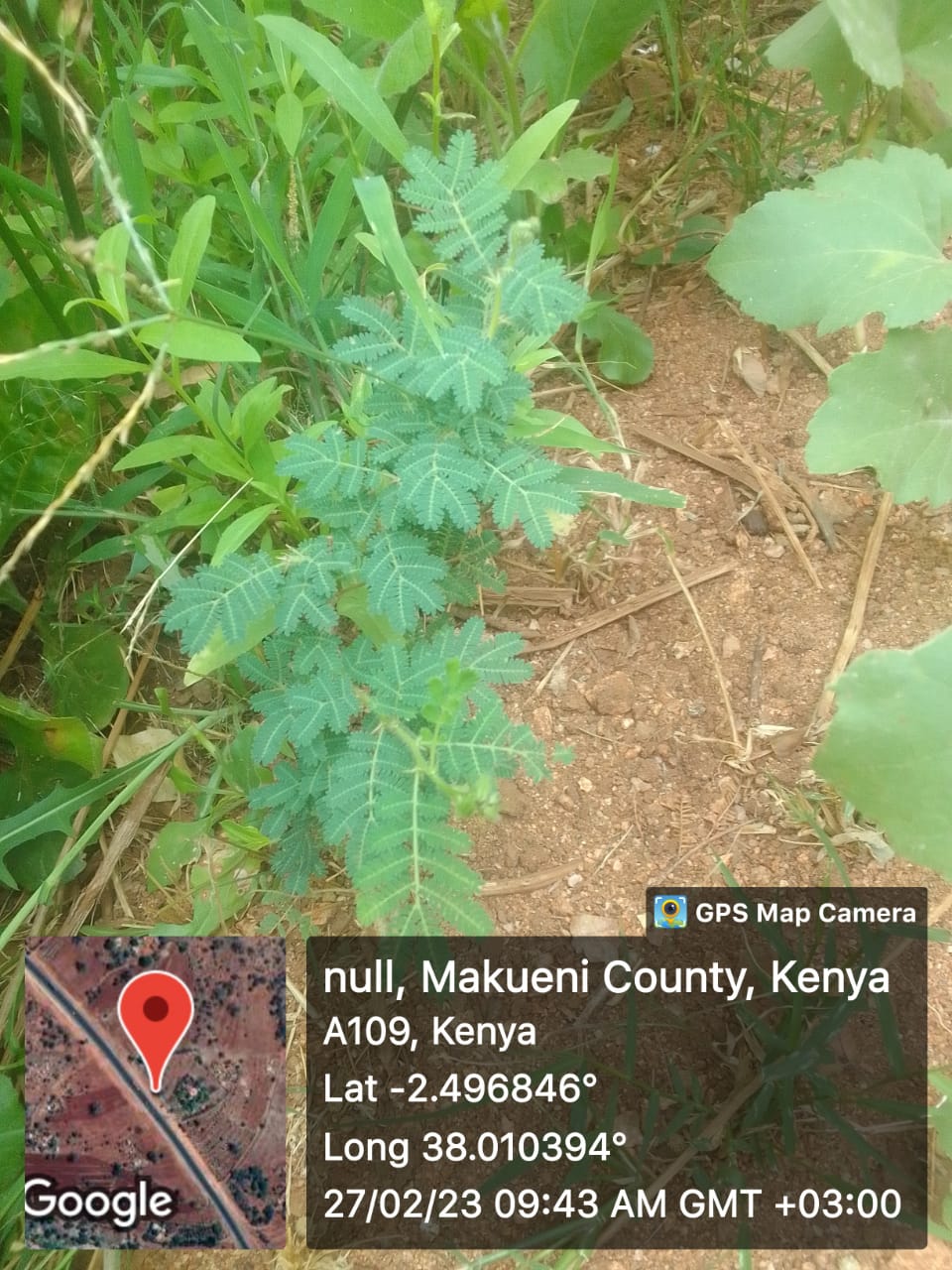This photo, captured using a GPS map camera, presents a top-down view of lush green leaves and shrubbery growing from the ground, interspersed with elements of dirt and grass. The primary focus of the image is a distinct plant emerging prominently from the foliage. At the bottom of the photo, two informational boxes provide context to the scene. The left box displays a Google Maps pin, marking the exact location of the photograph. The right box, with a transparent background, includes detailed geographical information: "Mukuni County, Kenya," along with precise coordinates of latitude -2.496846 degrees and longitude 38.010394 degrees. The timestamp at the bottom right corner indicates the picture was taken on February 27, 2023, at 9:43 AM GMT+3.